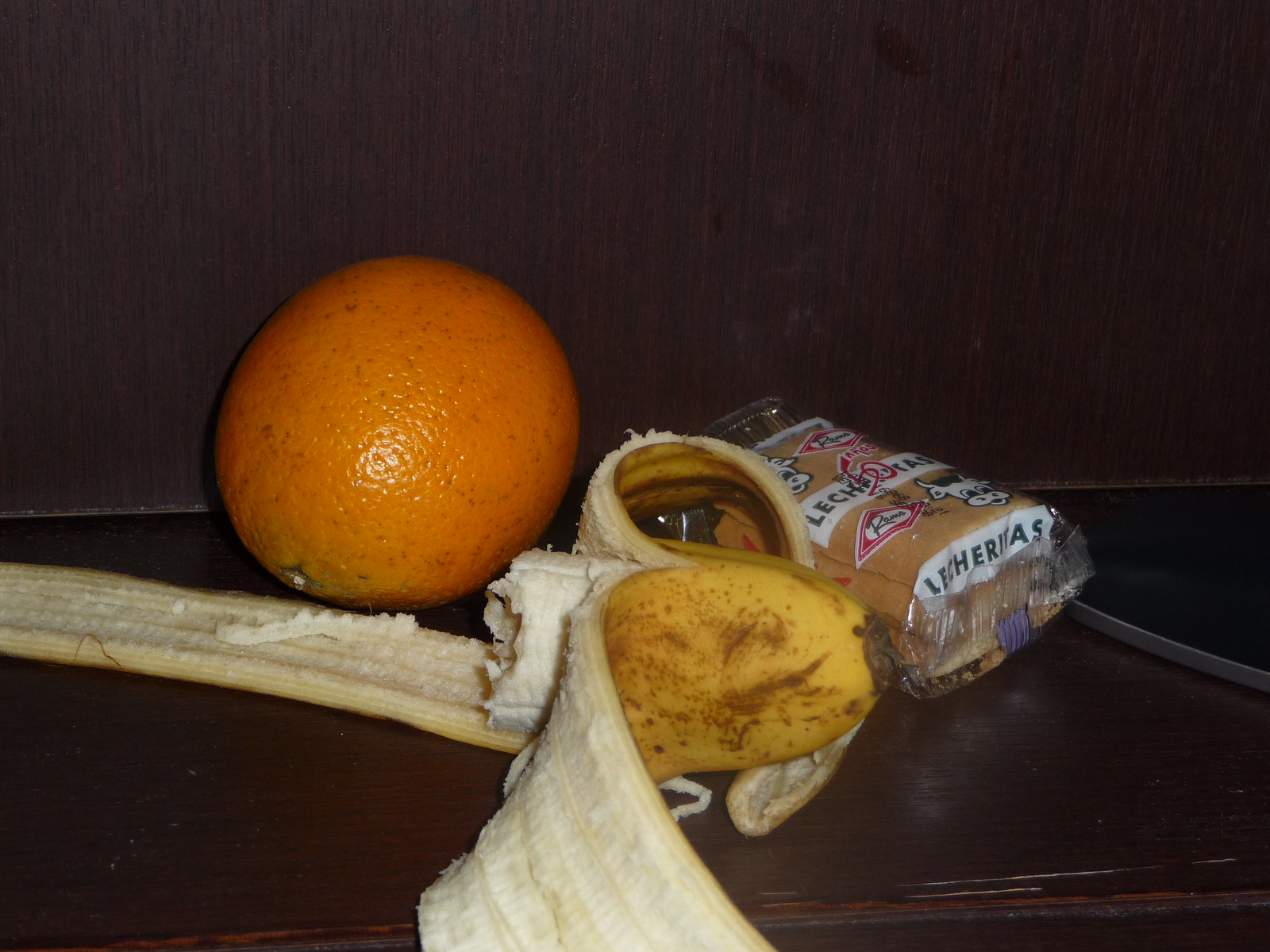This photograph showcases an assortment of food items artfully arranged on a dark brown wooden surface. To the left, an orange is positioned at a tilt, catching a glint of light that draws attention to its textured rind. Centrally located in the composition is a partially peeled and half-eaten banana, its peel cascading forward and resting gently in front of the orange. To the right and slightly behind the banana peel, a soft cookie or pastry remains enclosed in its packaging, which features a colorful cartoon cow and a distinctive red logo and red lettering. The packaging's side, adorned with black letters on a white background, reads "Le Charitas." The entire scene is set against a backdrop of dark brown paneling, enhancing the rustic and cozy atmosphere of the image.